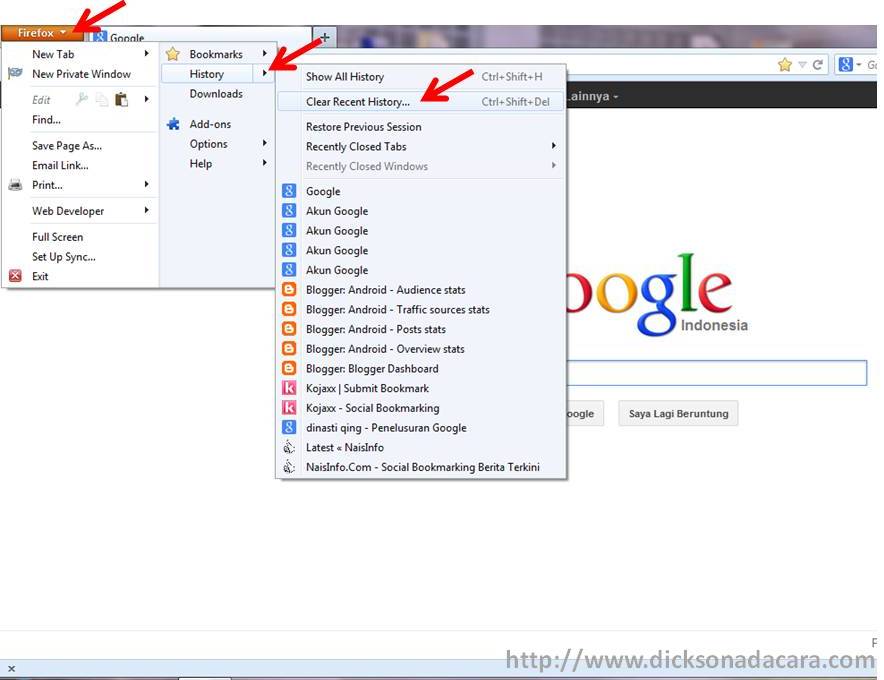A detailed screenshot displays a user navigating through the Firefox browser menus. The left side of the screen showcases several tabs, with Google open and displaying a search page localized to Indonesia. The primary Firefox menu is expanded, revealing options such as 'New Tab,' 'New Private Window,' 'Save Page As,' 'Email Link,' 'Print,' 'Web Developer,' 'Full Screen,' 'Set Up Sync,' and 'Exit.' 

A red arrow highlights the 'History' option within this menu, and there is an additional red arrow pointing towards the sub-menu that appears when the History option is selected. This sub-menu features several options including 'Bookmarks,' 'History,' 'Downloads,' 'Add-ons,' 'Options,' and 'Help.'

Within the expanded History sub-menu, the option 'Clear Recent History...' is second from the top and is marked with another red arrow. The screenshot details many of the user's recent activities, showing a mix of Google search results, blog visits, and other browser activities with approximately 10-15 listed entries.

Overall, this screenshot serves as a tutorial on how to access and clear your browsing history in Firefox. The bottom of the image contains the website URL: http://www.dixonadakara.com.